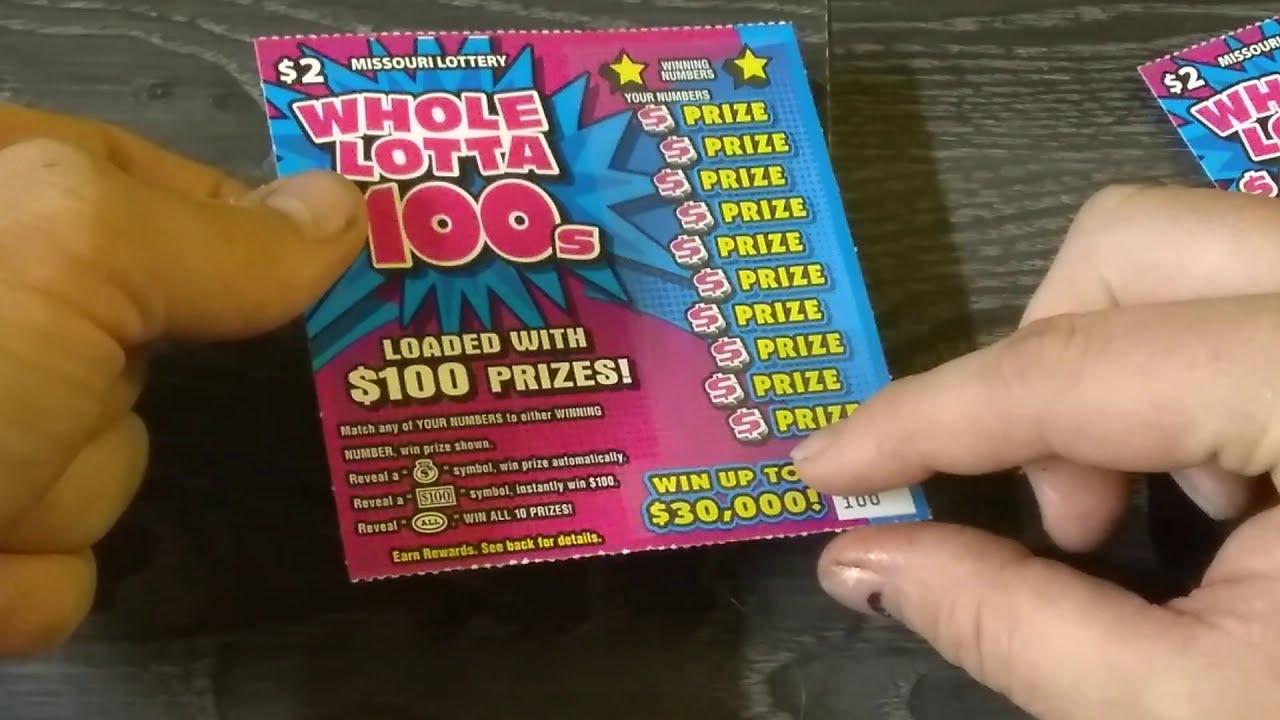In this close-up image, a pair of hands with a light tan complexion are holding a pink Missouri Lottery ticket titled "Hole Lotta 100s." The ticket costs $2. The left hand grips the ticket near the top, while the right hand points to the text stating "Went up to $30,000" at the bottom. The ticket rests on a gray wooden surface, with a visible seam where two planks meet. The ticket features a dynamic blue explosion graphic in the top-left corner with the title "Hole Lotta 100s" written in pink over the blue. The words "Loaded with $100 Prizes" are printed below the title. On the right side, a column of text reads "Prize" repeatedly, adjacent to the flap-covered "Your Numbers" section. Other notable details include two vertical yellow stars and instructional text about matching numbers to win. In the upper right corner of the image, part of another lottery ticket is visible.